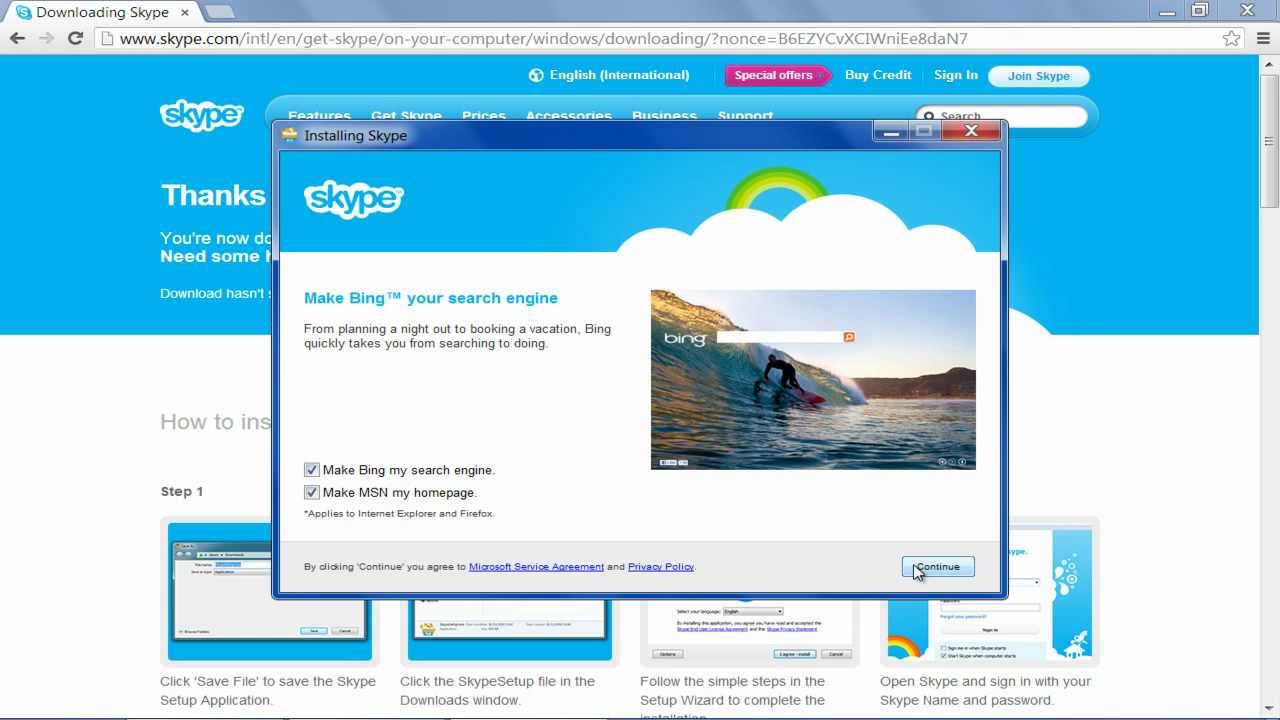This image captures a computer monitor displaying the Skype.com website. The browser's gray tab in the upper left corner indicates the activity of "downloading Skype," while the URL bar below confirms the user is on Skype.com, presenting a personalized link. The familiar horizontal blue banner of the Skype website is prominently featured at the top, adorned with the recognizable Skype logo in blue and white in the upper left corner.

A prominent pop-up window occupies a significant portion of the screen. This pop-up promotes setting Bing as the default search engine with the phrase: "Make Bing your search engine from planning a night out to booking a vacation," and features an image of a Bing homepage. The pop-up includes checkboxes for "Make Bing your search page" and "Make MSN your home page," both of which are checked off. The mouse cursor is poised over the blue "Continue" button in the bottom right corner of the pop-up, suggesting imminent user action.

At the very bottom of the page, four small thumbnails illustrate the Skype installation process, though only partially visible due to the overlay of the pop-up. On the left side of the pop-up, a fragment of the phrase "how to install" is discernible. The four thumbnails provide a step-by-step visual guide with text beneath each image, instructing users to: "click save file to save the Skype setup application," culminating in the final step of "open Skype and sign in with your Skype name and password."